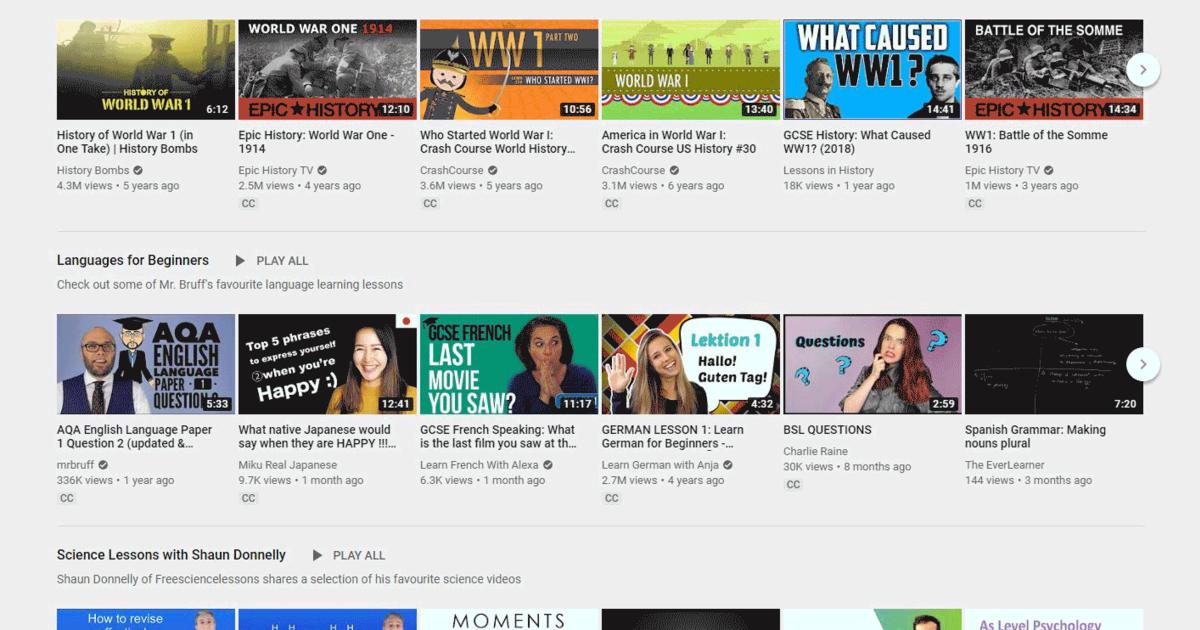This screenshot captures an old version of YouTube's homepage, likely from before 2020, characterized by its distinct material design layout and a light gray background instead of white. The page is divided into multiple sections, with three visible segments.

The first partially visible section appears to focus on videos about World War I history. The second section is titled "Languages for Beginners" and includes a variety of educational videos covering different languages. Notable video titles include "AQA English Language Paper 1," "What Native Japanese Should Say When They Are Happy!" and tutorials on French, German, and ESL (English as a Second Language). Additionally, there is a video on Spanish grammar titled "Making Nouns Plural."

The final segment at the bottom of the page features "Science Lessons with Sean Donnelly." However, the full details of these videos are cut off and not discernible from the screenshot.